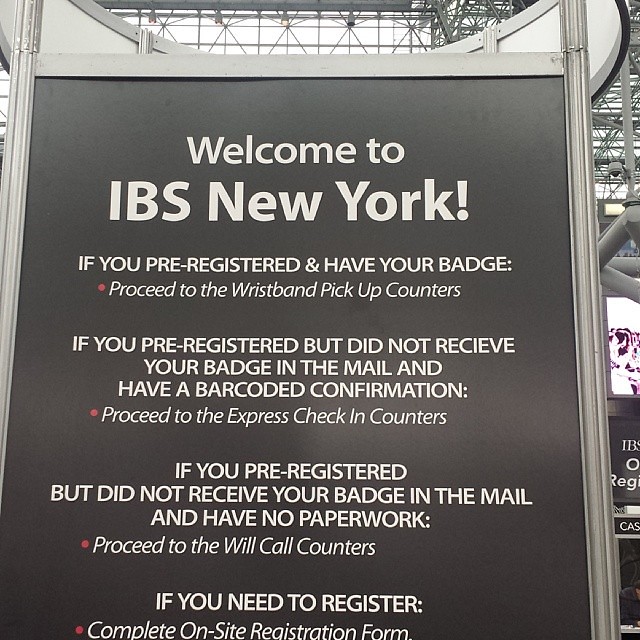A striking black sign or plaque, adorned with a sleek, chrome metal border, commands attention. On the black background, white text prominently displays a welcoming message: "Welcome to IBS New York." Below this, a series of instructions are laid out, each prefaced by a red bullet point:

- If you pre-registered and have your badge, proceed to the wristband pickup counters.
- If you pre-registered but did not receive your badge in the mail and have a bar-coded confirmation, proceed to the express check-in counters.
- If you pre-registered but did not receive your badge in the mail and have no paperwork, proceed to the will call counters.
- If you need to register, complete an on-site registration form.

In the background, the hazy outline of a ceiling or scaffolding comes into view, marked by numerous criss-crossing metal bars, adding an industrial feel to the setting.